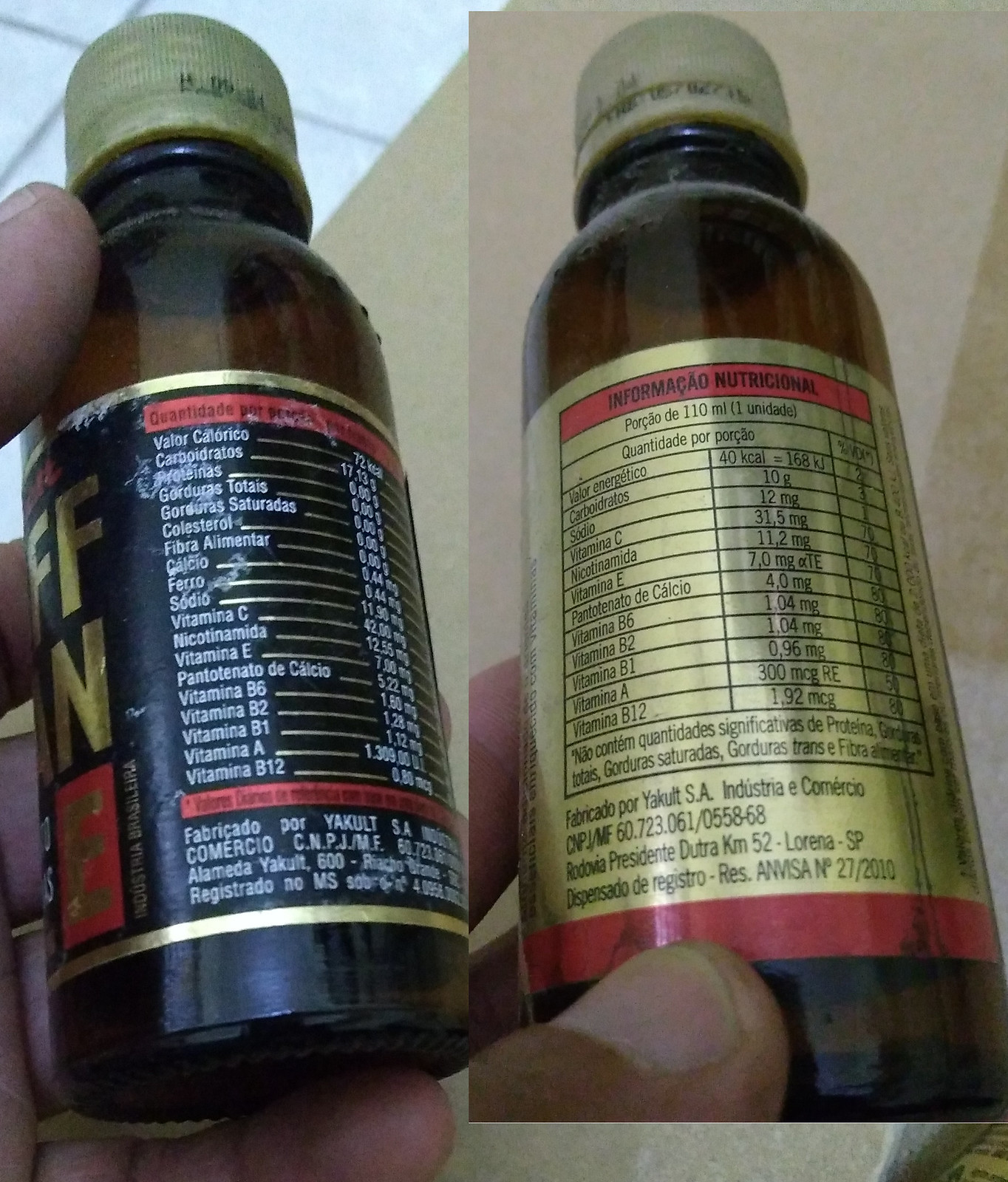A meticulously composed indoor photograph is split into two sections, showcasing the dual focus of the image. In one part, the photographer is seen dexterously holding an intriguing bottle in one hand while capturing the image with the other. The composition draws the viewer’s attention to the bottle, which is the focal point of the photograph. 

The bottle, held with care, stands out in its rich, dark brown hue, adorned with a sophisticated label in black, gold, and red. A gleaming gold cap sits atop, adding a touch of elegance. The label features text in Spanish, prominently displaying "Información Nutricional", indicating nutritional information. The intricate label also includes various details depicting vitamins and other attributes of the bottle's contents.

The background of the image is a serene combination of tan and white, likely the ground, adding a contrasting simplicity that highlights the bottle's allure. The careful balance and focus of the photograph emphasize the importance and details of the bottle, making it a captivating visual study of the object.